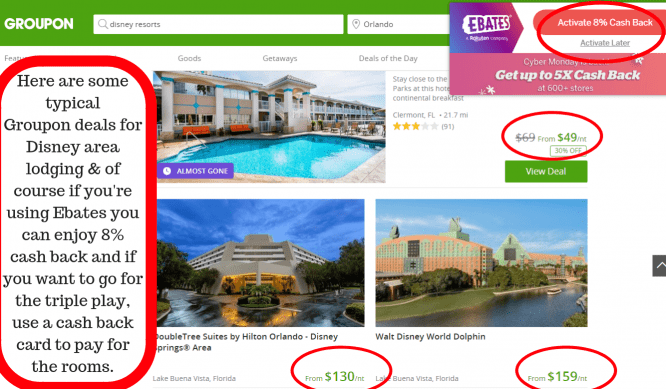The image displays a Groupon webpage featuring deals for Disney area lodging. Dominating the top of the page, a gray navigation bar spans across with the word "Groupon" prominently displayed in white on the left upper side. Below the navigation bar, the search field shows "Disney Resorts" with "Orlando" entered as the search query. An Ebates pop-up advertisement, purple with a white illustration, overlays part of the screen, offering 8% cash back with options to activate now or later.

On the left sidebar, it highlights, “Here are some typical Groupon deals for Disney area lodging,” and mentions that using Ebates could yield an additional 8% cash back. It also advises using a cash back card for maximum savings. 

The primary focus of the page is a vibrant image of a hotel room with a blue pool visible below. A small purple tag near the bottom of the image reads “Almost gone.” Below this image, a price drop is circled in red, showing a reduction from $69 to $49 alongside a green “View Deal” button.

Listed underneath are two more lodging options:
1. **DoubleTree Suites by Hilton Orlando, Disney Springs Area** - Highlighted with a red circle indicating a starting price of $130.
2. **Disney World Dolphin** - Also highlighted in red with prices starting from $159. 

The overall design effectively combines bright colors and strategic circles to emphasize attractive deals for potential travelers.